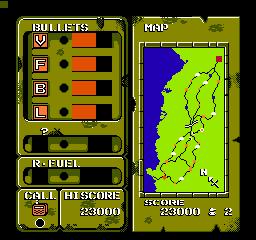This screenshot from a retro NES video game showcases an elaborate, olive-green and black menu screen typical of 8-bit artwork. On the top left corner, there are panels displaying four types of bullets labeled V, F, B, and L, reflecting different ammunition levels in orange. Beneath this, another box shows a question mark and 'R Fuel', indicating resources or fuel level. At the bottom left, a "Call" button and a high score counter proudly display a score of 23,000. Dominating the right side of the screen is a detailed map marked with various points, including three paths leading to a red square destination, complete with a compass to assist navigation. The menus feature a skeuomorphic design, reminiscent of metal, enhancing the retro aesthetic. This organized user interface appears to support a shooter game, possibly similar to titles like Guerrilla Warfare, combining tactical planning with arcade action.